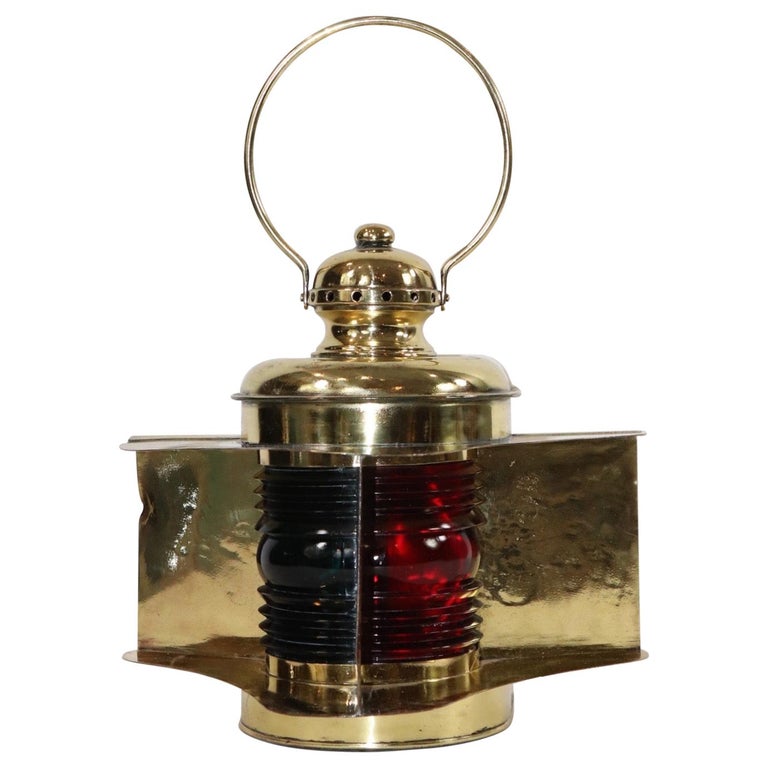The image depicts an antique brass lantern with a unique and detailed design. The lantern features a rounded, circular shape and a golden-brass body with a small handle for easy carrying or hanging. The lantern's glass bulb is divided into two distinct sides, each reflecting and amplifying light: the left side showcases a ridged, dark blue glass, while the right side presents a smooth, red glass. The top of the lantern has several ventilation holes, indicating functionality that either heat pushes out fumes or gaseous material. This dual-colored glass and reflective brass construction suggest it was perhaps used either as a light source or possibly for burning substances to ward off insects or create scent. The lantern, reminiscent of an old police lantern from the 1800s, stands out dramatically against the plain white gradient background, highlighting its intricate and timeless design.